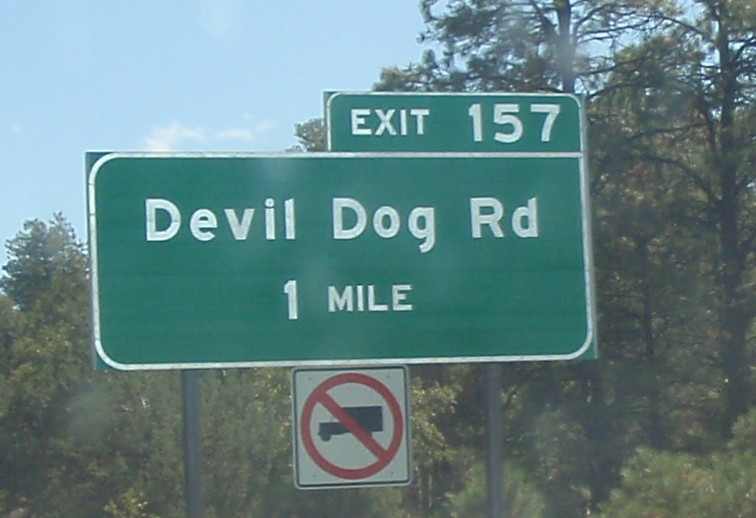This photograph captures a detailed view of a roadside sign along a highway, flanked by a lush forest and set against a pale blue sky with wispy clouds. The sign prominently features a large green rectangular panel with a white border, displaying "Devil Dog Road 1 mile" in bold white text. Above this panel is a smaller green rectangular sign, about half the width of the main sign, which reads "Exit 157" in white lettering. Below the large sign is a smaller white square sign with a black border, featuring a black silhouette of a truck crossed out by a red circle with a diagonal line, indicating that trucks are prohibited on this road. The entire sign assembly is supported by two poles. Visible in the background are dense, green trees, adding a scenic, wooded backdrop to the signage. The image also hints at imperfections on the car window from where the photo was taken, such as smudges or reflections.